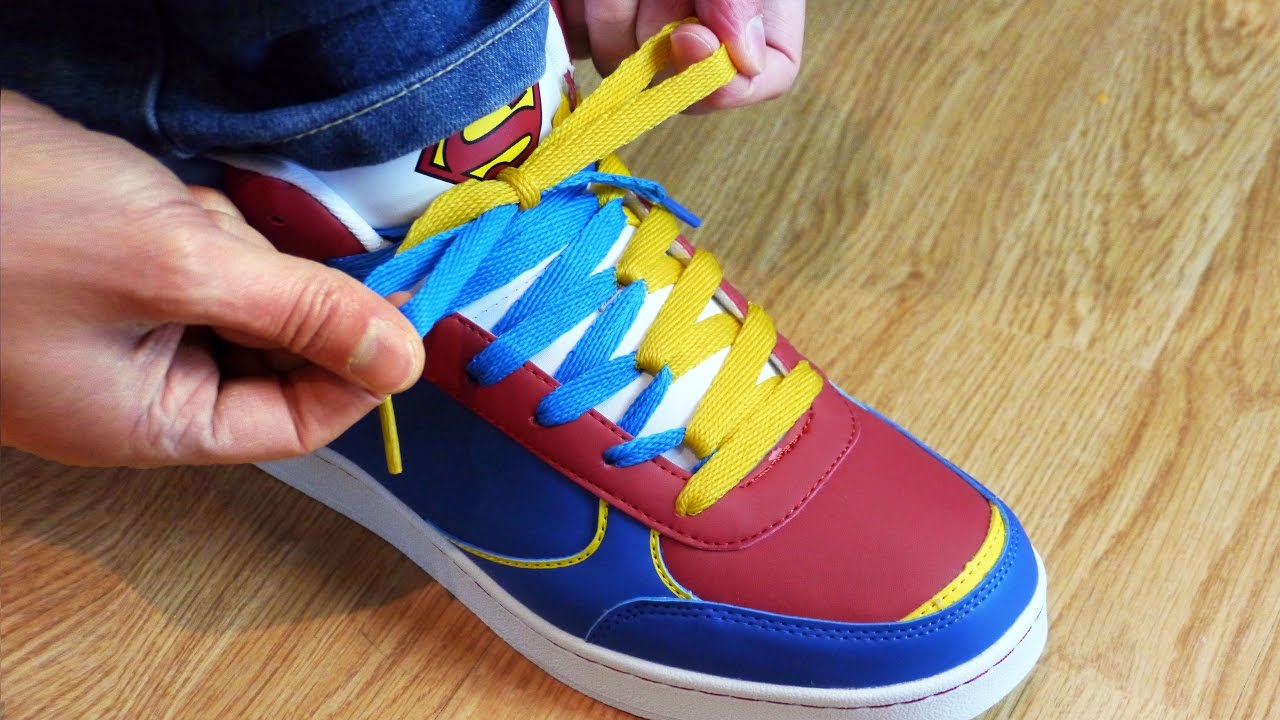In a full-color, horizontally rectangular photograph with no borders, we observe a staged indoor scene lit by artificial light. The background features a light-grained wooden floor with visible grains and knots. Central to the image is a children's tennis shoe, which prominently displays the red and yellow Superman logo on its tongue. The shoe is a vibrant mix of red, yellow, and blue, with additional white detailing. The laces are a combination of blue and yellow, crossing over one another as they are tied. The lower part of a pair of blue jeans with yellow stitching is partially visible, alongside two Caucasian adult male hands that are busy tying the shoe. The scene emphasizes the adult's hands attending to the child's shoe, highlighting the care and attention being given.